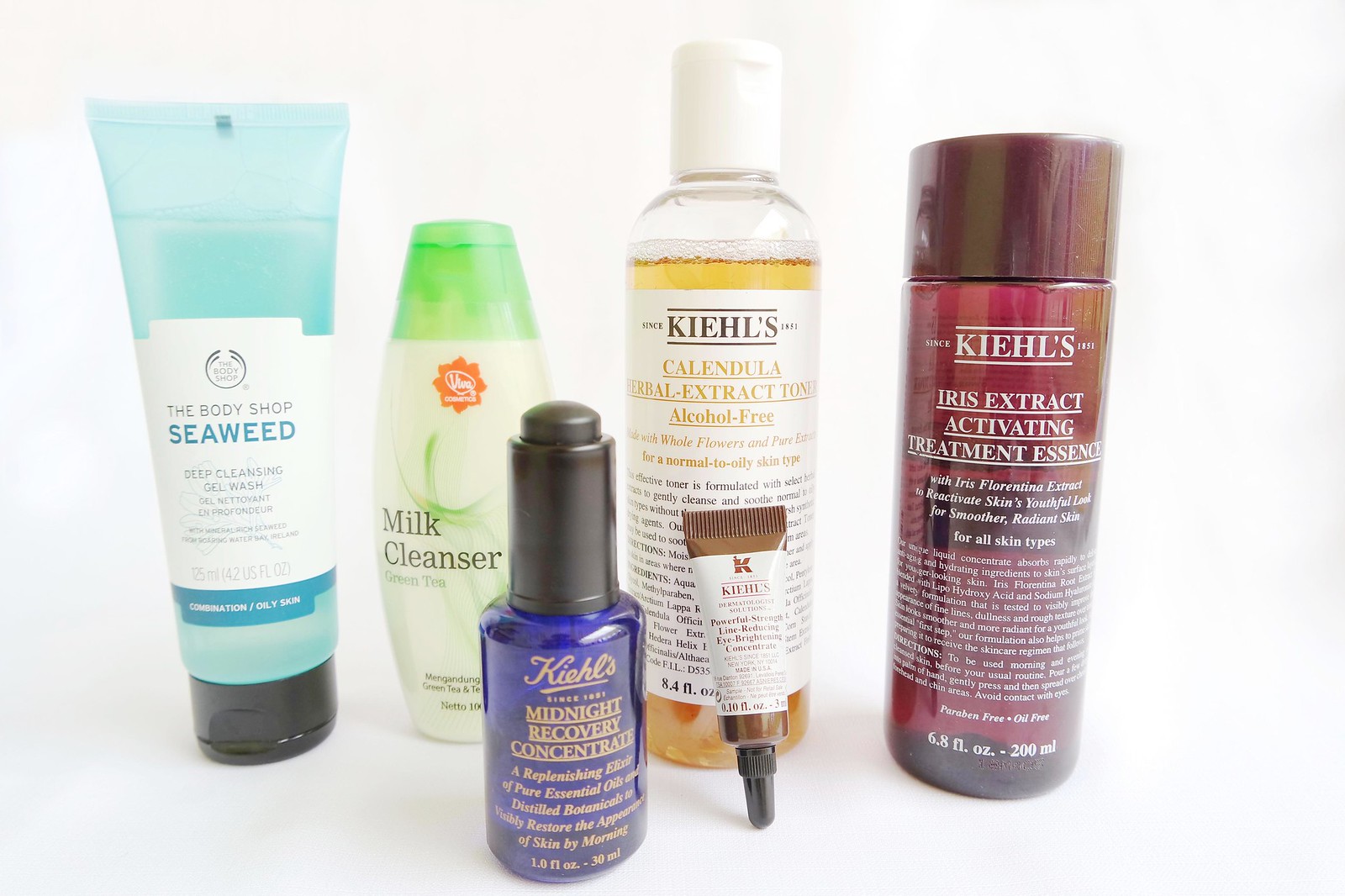In this studio-shot image, we see a meticulously arranged collection of skincare products against a pristine white backdrop, showcasing each item with exceptional lighting quality that highlights their details. On the left, there is a blue bottle labeled "Body Shop Seaweed Deep Cleansing Gel Wash" designed for combination and oily skin. Next to it stands a green tube named "Milk Cleanser Green Tea." Positioned nearer to the camera is a blue dropper bottle that reads "Midnight Recovery Concentrate," described as a replenishing elixir of pure essential oils and distilled botanicals, promising to visibly restore the appearance of skin by morning. Adjacent to this is a bottle of "Calendula Herbal Extraction Toner," which is alcohol-free. Leaning against the toner is a small tube of "Powerful-Strength Line-Reducing Eye-Brightening Concentrate." Lastly, we see a dark red bottle labeled "Iris Extract Activating Treatment Essence," which is suitable for all skin types. The carefully curated placement and high-quality image capture work together to emphasize the variety and purpose of each product in the lineup.